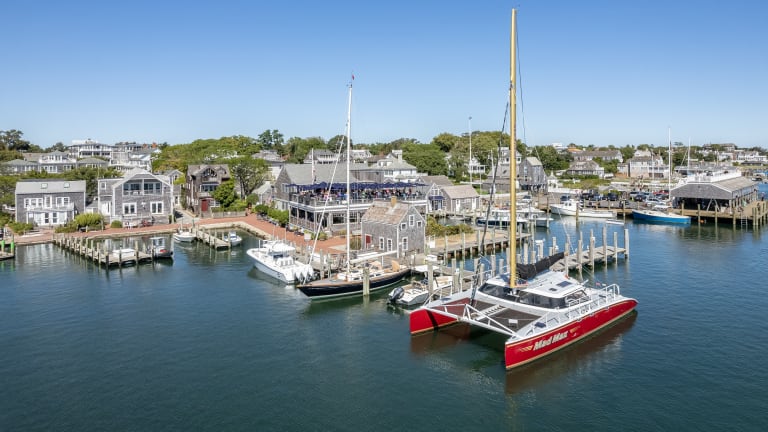The photograph captures a vibrant aerial view of a coastal harbor town under a slightly hazy but sunlit blue sky. The vivid blue water reflects the boats and piers, enhancing the picturesque scene. Along the shore, a variety of light gray and white-trimmed buildings, mostly two-story and possibly on stilts, are interspersed with lush green trees. A brown boardwalk with numerous piers and docking posts meanders along the water’s edge. At the center of the boardwalk, a significant structure stands out, likely a large restaurant with a second-tier deck adorned with blue umbrellas.

In the harbor, several boats are moored, including various sailboats, motorboats, and yachts. Notably, a large catamaran with a wide enclosed cabin, two red pontoons, and a high mast is prominent in the foreground. Nearby, a red and white sailboat with a gold mast, another sailboat, and a white yacht add to the bustling maritime activity. Further in the distance, a blue fishing boat and another white yacht can be seen. The serene scene is completed by the reflective water and the clear blue sky, making it a quintessential representation of a lively port town.